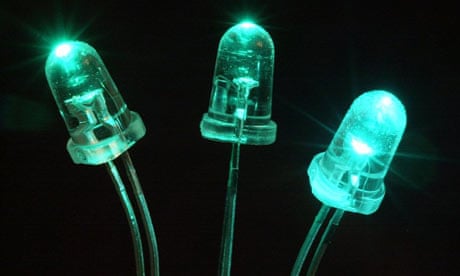This photograph is a dramatic close-up of three glowing blue LED lights set against a solid black background. Each LED is encased in a translucent, dome-shaped cap through which the internal components are visible. The first LED, positioned on the left, curves slightly to the left, featuring a bright tip emitting a small white spot with rays of light radiating from it. The second LED in the middle is nearly vertical but tilts slightly to the right, shining brightly with two distinct white spots where the brightness peaks. The third LED on the right curves to the right and is similarly bright, showcasing a bluish-green aura at its tip. All three LEDs emit a striking blue light that lightly illuminates the wires emerging from their dome-shaped caps. The background remains uniformly black, highlighting the vivid blues and subtle aqua hues of the LEDs while a delicate starburst pattern emanates from each light, creating an ethereal and captivating visual effect.